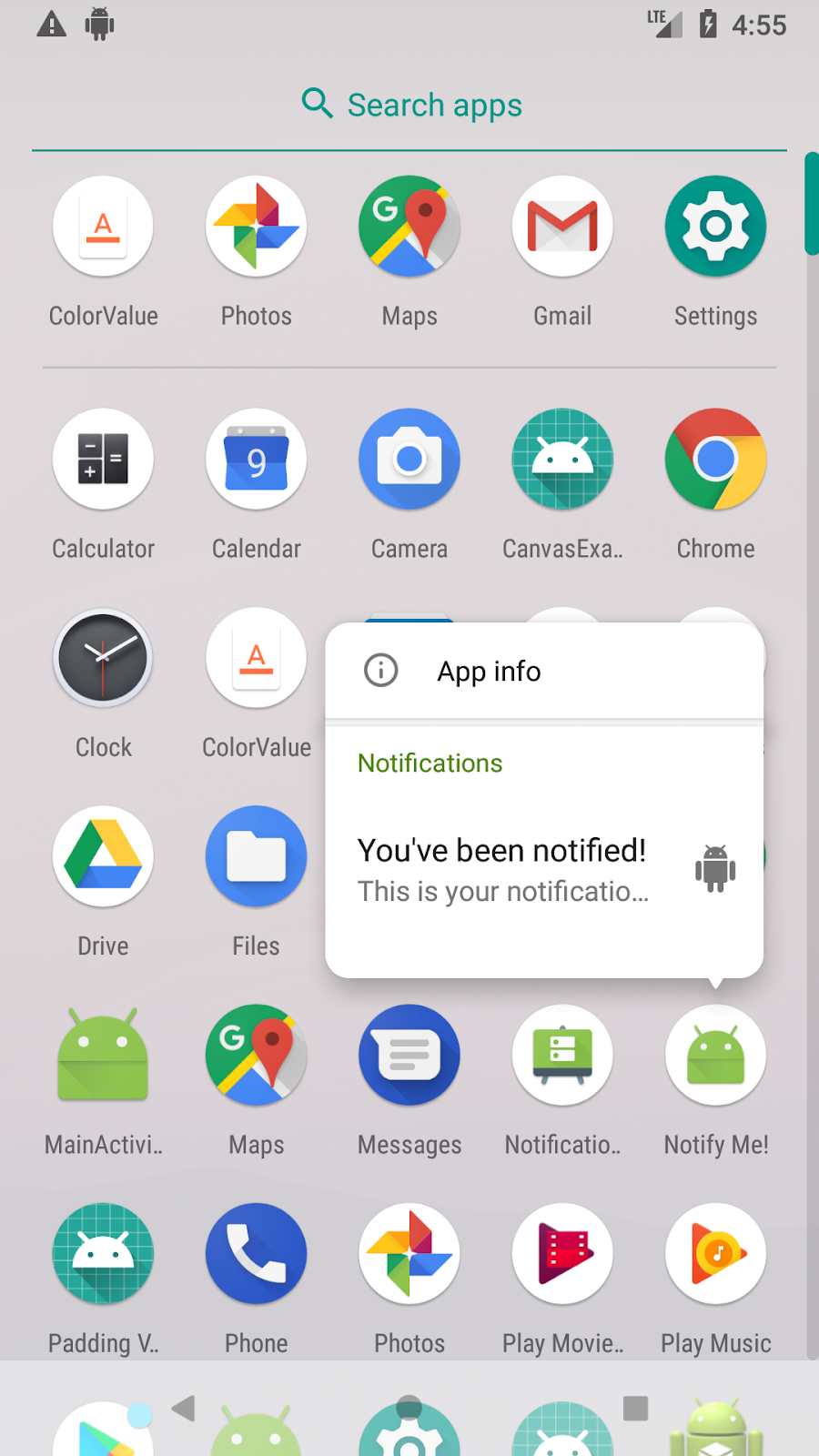**Detailed Caption**

This image is a portrait-oriented screenshot of a smartphone displaying the "Search Apps" function. At the top-left corner, there is a grey triangle with a white exclamation mark, and next to it, a robot icon. Across the top-right of the screen, the status indicators show "LTE" with a half-filled signal icon resembling a mountain, a fully charged battery marked by a black battery icon with a white lightning bolt, and the time displayed as 4:55. The background of the screen is grey.

Below these top icons, there is a green magnifying glass icon and the text "Search apps" also in green. A horizontal line stretches across the screen beneath this search bar. The main part of the display features a grid of app icons arranged in five columns and seven rows.

- **Top Row (from left to right):**
  1. **Color Value**: White background with an orange "A" and an orange underline.
  2. **Photos**: White background with yellow, red, blue, and green rhomboidal shapes forming a circle or square.
  3. **Maps**: Typical Google Maps icon.
  4. **Gmail**: White background with a red "M".
  5. **Settings**: Green background with a white cog.

- **Second Row:**
  1. **Calculator**: White background with a red "+" (black outline), a white "-" (black outline), and a white "=" (black).
  2. **Calendar**: Blue flip calendar icon with the number "9".
  3. **Camera**: Blue background with a white camera and a blue lens.
  4. **Canvas EXA**: Green and white graph paper background with a white robot head with two antennae.
  5. **Chrome**: Red, green, and yellow circle with a blue center.

- **Third Row**: 
  1. **Clock**: Black background showing the time as 10:10 with a red second hand and white hour and minute hands.
  2. **Color Value**: Same as in the top row.
  3. **Three icons blocked by a pop-up**.

- **Fourth Row**: 
  1. **Drive**: White background with a yellow, blue, and green triangle.
  2. **Files**: Blue background with a white file icon.
  3. **Three more icons blocked by the pop-up**.

- **Fifth Row**: 
  1. **Main Activity**: Green robot with two antennae and white eyes.
  2. **Maps**: Same as mentioned before.
  3. **Messages**: Blue background with a white speech bubble.
  4. **Notifications**: White background with what appears to be a green chest of drawers or filing cabinet.
  5. **Notify Me**: White background with a green robot head.

- **Sixth Row**: 
  1. **Padding V**: Green and white graph type background with a white robot head.
  2. **Phone**: Blue background with a white handset icon.
  3. **Photos**: Same as mentioned earlier.
  4. **Play Movies**: White background with a red triangle and red ticket.
  5. **Play Music**: White background with an orange triangle and concentric circles in yellow and orange with a white center.

There is also a bottom row of app icons, partially visible but too small to identify specific details. However, it includes icons that resemble the Google Play Store, Main Activities, Settings, another robot on a graph background, and the green robot seen earlier but showing more of its body.

In the center, obscuring parts of the third and fourth rows, there is a white pop-up notification. The pop-up reads "App Info Notifications: You've been notified. This is your notification" in a white text box. A grey alien icon accompanies this notification.